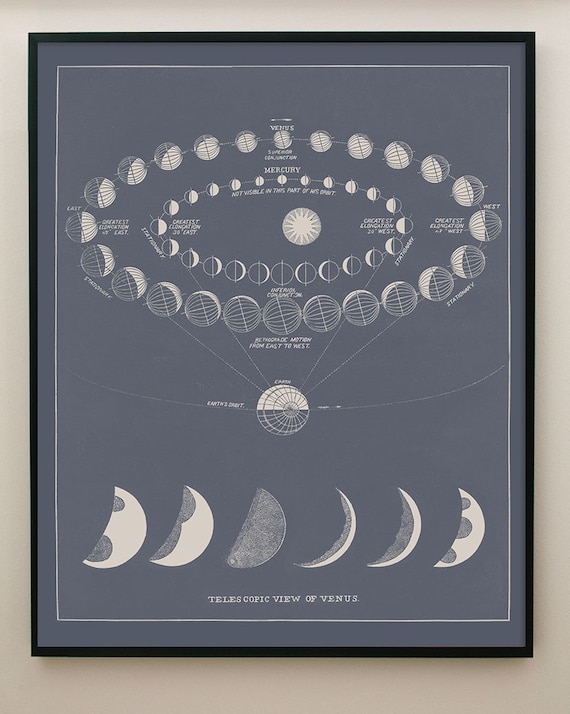The framed poster, hanging on a beige wall, presents a fascinating depiction of celestial bodies and their phases. Encased in a thin black frame, the poster features a dark grey background with a white border along the edges. At the top, there is a detailed image of a full moon. Surrounding this central moon, there are two concentric rings of smaller spheres, with the outer ring consisting of larger spheres and the inner ring showcasing smaller ones. The inner circle represents the planet Mercury, labeled with phrases such as "not visible in this part of the orbit" and "stationary." The outer circle displays the planet Venus. The very center of the inner circle showcases the Sun. Additionally, across the bottom of the image, there are multiple crescent shapes depicting different telescopic views of Venus with some accompanying text that is difficult to read. This layered representation intricately combines elements of both the moon's phases and planetary orbits.